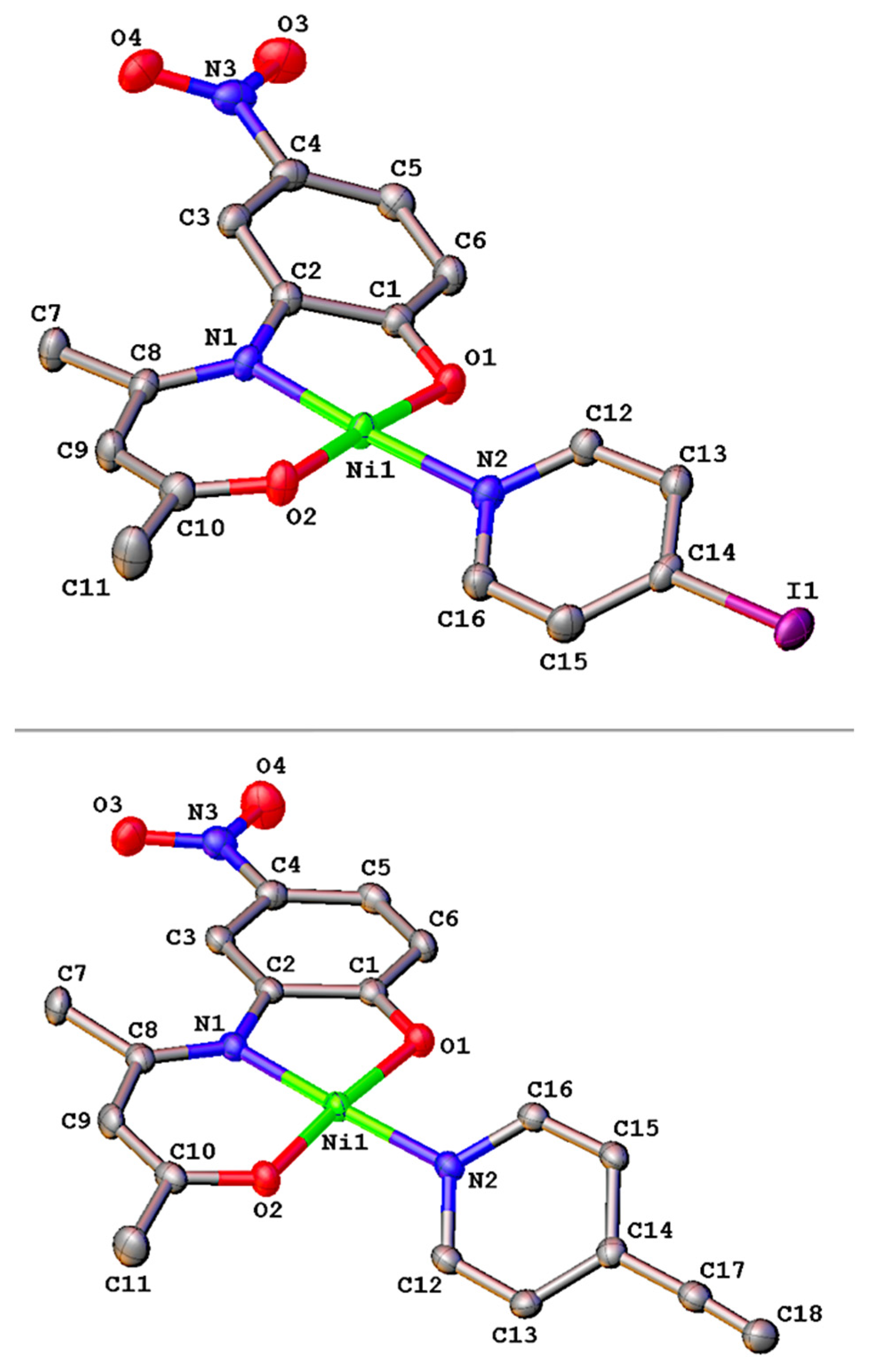The image presents a pair of digitally rendered scientific charts, positioned one above the other, occupying the entire frame. Each chart illustrates complex molecular structures, resembling chemical bond representations or DNA strands. Both charts feature labeled segments with letters and numbers: annotations like O4, N3, O3, C1 through C16, and NI1. The elements appear color-coded—oxygen atoms are symbolized by red, nitrogen by blue, carbon by gray, and nickel (NI) by green. The upper chart also includes a purple element labeled 'I,' which is absent from the lower chart. No legible text or keys are provided to explain the image, making its exact nature ambiguous. The color palette includes white, black, red, green, pink, and gray, suggesting an educational context, potentially an infographic detailing chemical compounds or molecular structures.